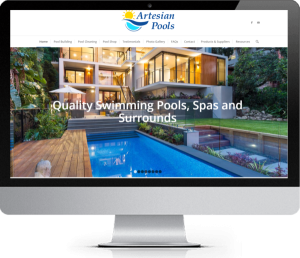A sleek, modern computer monitor with a stylish silver-gray pedestal and a prominent black bezel at the bottom is displayed. The bezel hosts a black strip that contrasts with the silvery-gray plastic of the monitor, matching the pedestal’s color. The screen showcases a web page titled "Artisan Pools." Although the text is somewhat small and difficult to read, the Artisan Pools logo is clearly visible at the top. Below the logo, there are several tabs or buttons that are not entirely legible. The central focus of the webpage is a captivating image of a magnificent mansion featuring a luxurious swimming pool. Accompanying the image is the text: "Quality swimming pools, spas, and surrounds," indicating that the webpage is likely an advertisement for Artisan Pools.